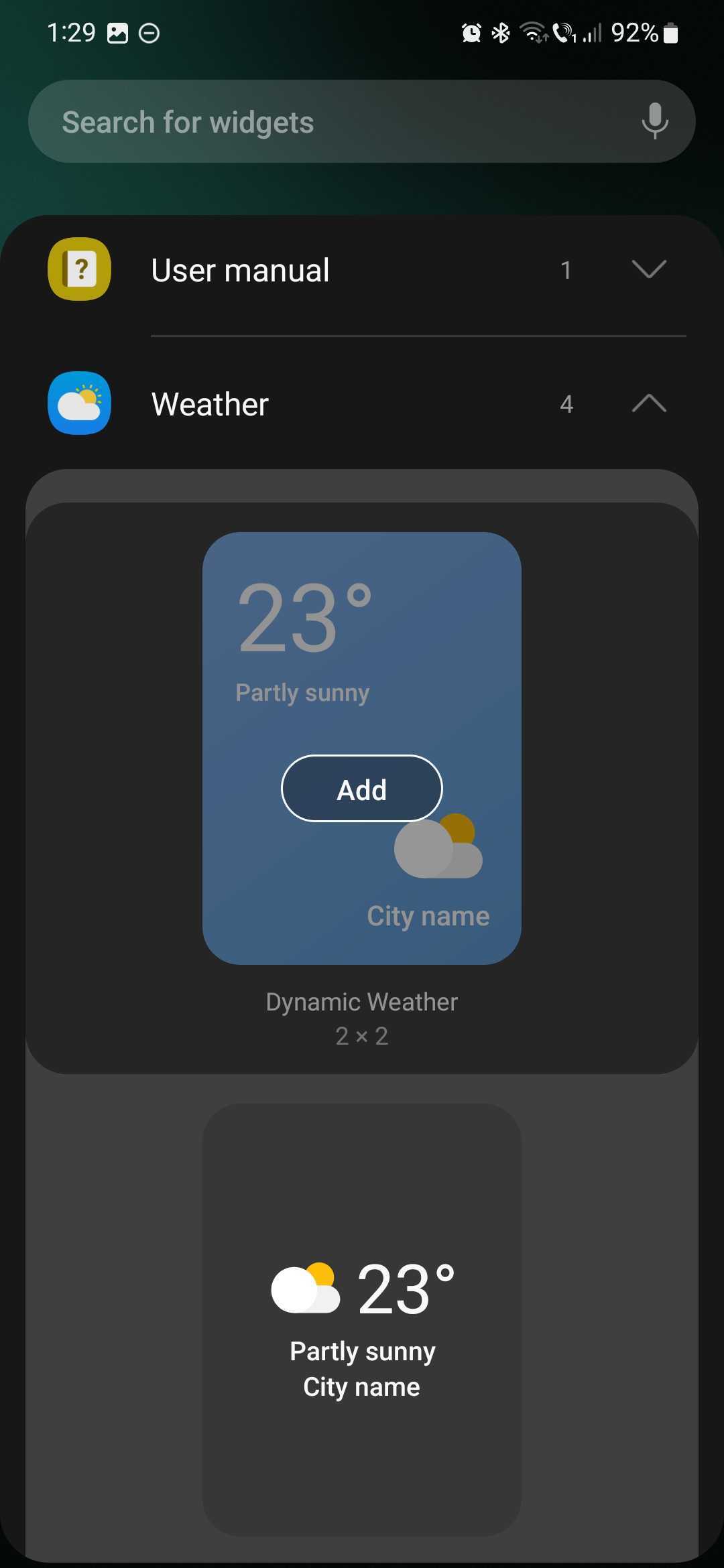The screenshot displays a smartphone interface with a predominantly black background. 

- **Top-left corner:** The time is displayed in white, followed by two icons.
- **Top-right corner:** Icons for an alarm, battery status, and reception are present.
- **Below the status bar:** A horizontal oval-shaped search bar reads "Search for widgets" on the left in white text. On the right side of the bar, there's a gray microphone icon.
- **Mid-section:** A black rectangle appears about three lines down. On its left is an oval with a mustard-colored background, featuring a beige square with a brown question mark in the center. To the right, in white text, it says "User manual." Further right, there is a light gray ellipsis (three dots) and a downward arrow resembling a "V."
- **Below the rectangle:** A blue weather icon with a cloud is visible, labelled "Weather" to its right. To its far right, there is a number "4" accompanied by an up arrow.
- **Lower section:** A light gray rectangle strip hosts a centered black rectangle. Inside the black rectangle, a blue square displays:
  - On the upper left, the number "23°" (degrees) in white.
  - Directly below, it says "Partly Sunny" in white.
- **Centered:** A dark gray "Add" button outlined in white, with "Add" written in white.
- **Lower right of the blue square:** An icon depicting a cloud with a sun on its upper right-hand side, labelled "City Name" in white.
- **Bottom of the box:** "Dynamic Weather" in white, followed by "2x2" in gray.
- **Bottom segment:** A darker gray square on a light gray background features a white cloud with a yellow sun (resembling a fried egg) in the center:
  - "23°" (degrees) in white below the icon.
  - "Partly Sunny" in white text.
  - Finally, "City Name" in white at the bottom.